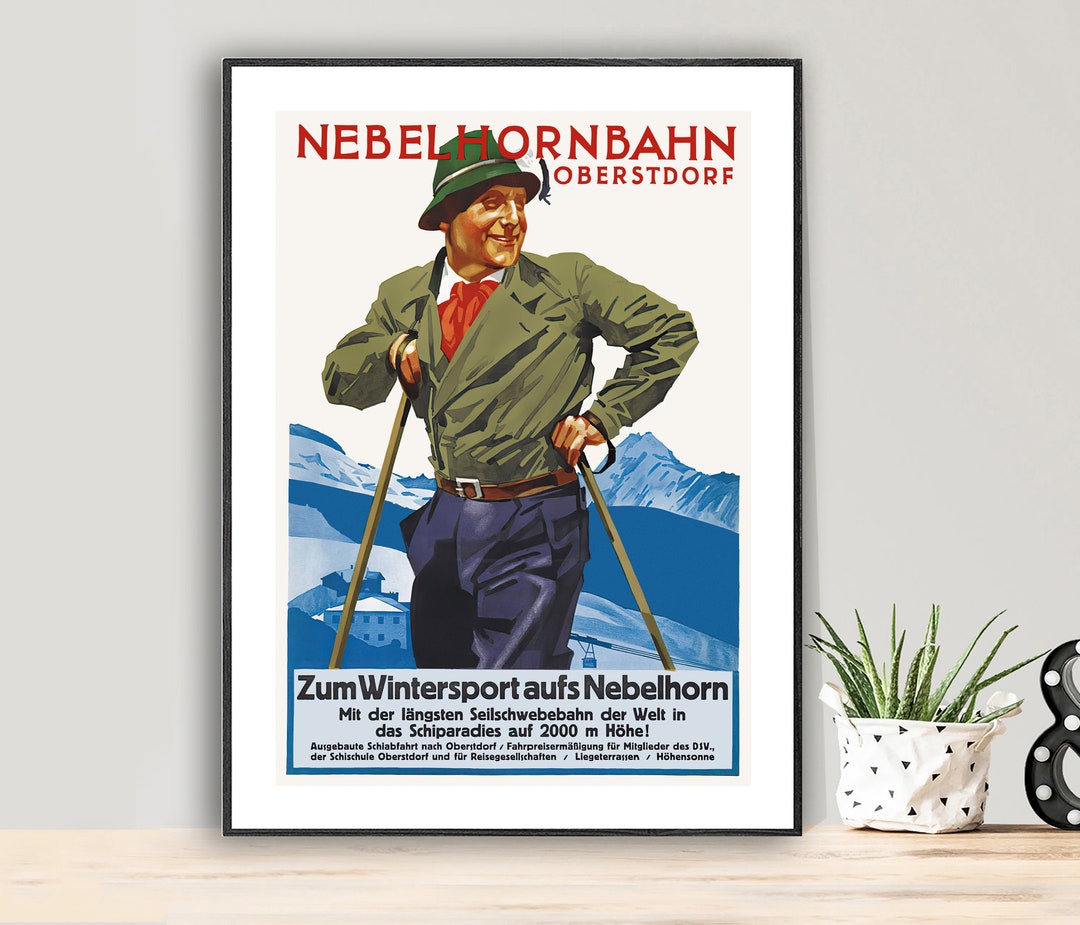In this computer-generated image designed to showcase art in a realistic setting, we see a framed vintage-style German poster displayed on a whitish-brown desk against a gray wall. The artwork, potentially an advertisement for winter sports, features a German soldier skiing against a backdrop of mountains, likely in Austria. The skier, depicted with a cheerful smile, wears an olive green jacket, a red scarf, a bright green hat, blue pants, and a brown belt, and holds ski poles in each hand. The text on the poster reads "Nebelhornbahn Oberstdorf" in red at the top and "Zum Wintersport am Nebelhorn" below, with additional German text in smaller font underneath. Enhancing the scene, a green plant with long stems, held in a white cloth decorated with black triangles, sits near the framed artwork, adding a touch of nature to the composition.